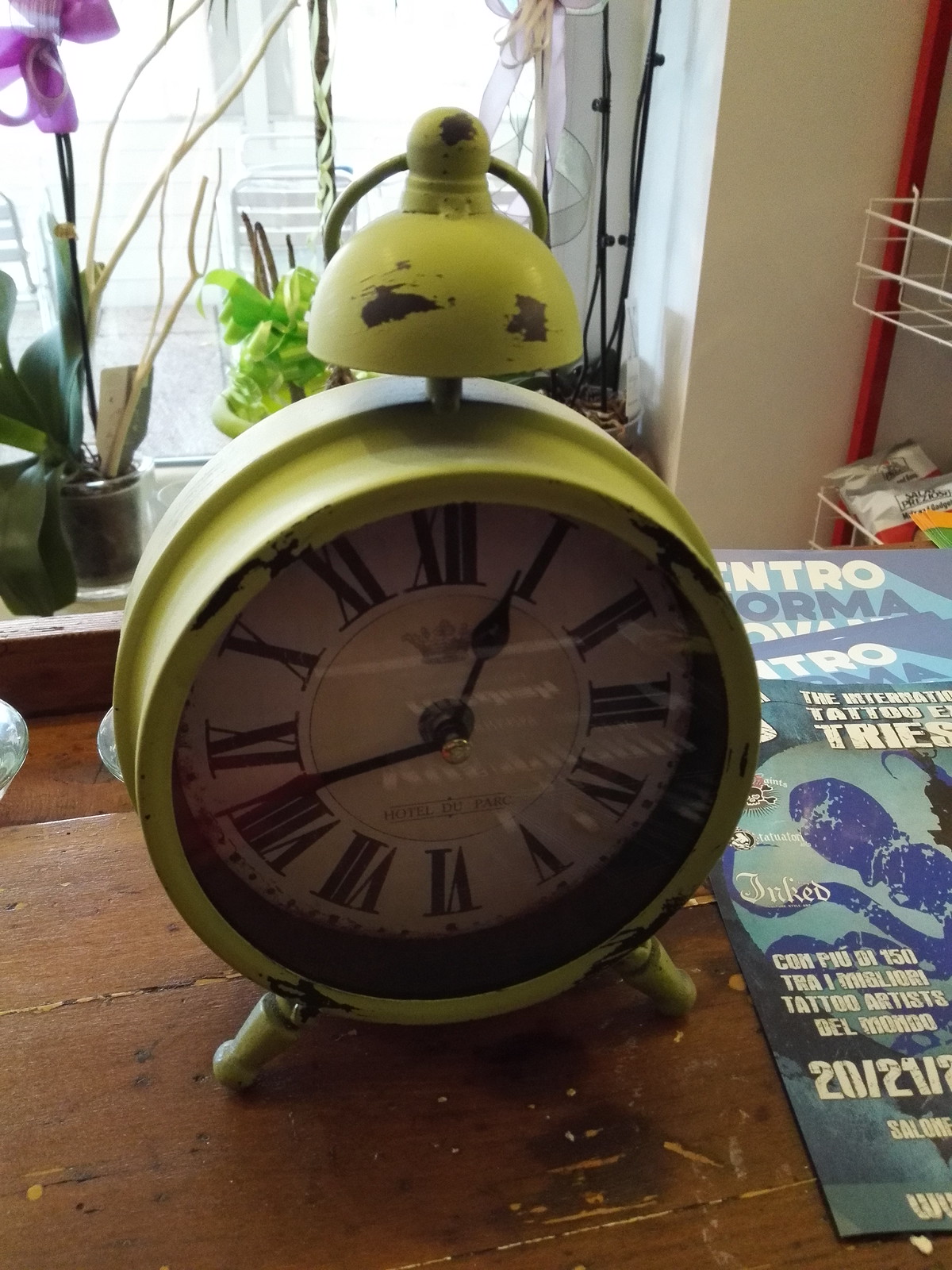A meticulously captured photograph showcases an old-fashioned alarm clock prominently placed on a wooden table or nightstand. The clock, adorned in lime green paint that is visibly chipped at both the top and bottom, features an antique face with Roman numerals set against a white background. The image is closely cropped, highlighting only small details of the surrounding environment. To the right of the clock lie two event or concert flyers, with only fragmentary text visible, including the word "inked." In the background, a window allows natural light to highlight a pink orchid with one bloom barely within the frame at the upper left corner. Adjacent to this, a small, indiscernible green plant adds to the eclectic assortment, and another orchid with white petals is subtly visible, largely cropped out of the frame. The scene evokes a sense of vintage charm mingled with the serenity of indoor plants.